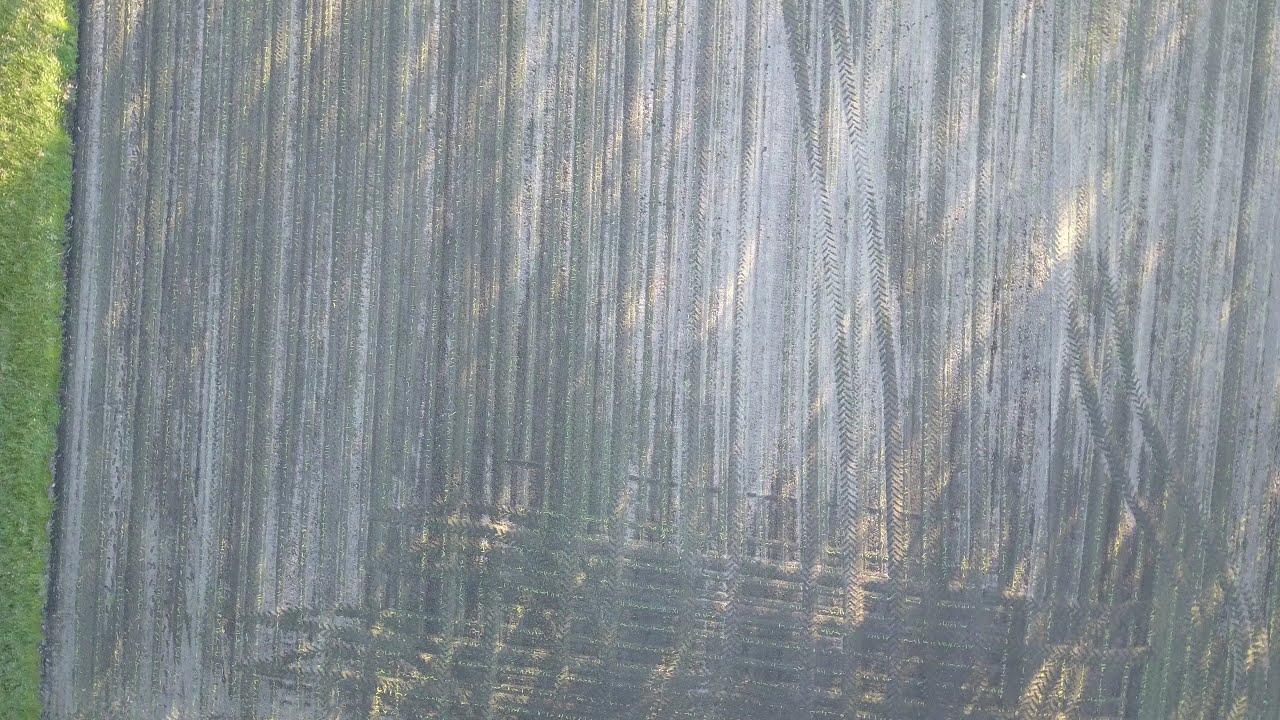In this image, which appears to be a close-up aerial or zoomed-in shot taken outdoors, the primary focus is on a vast gray surface that stretches across the frame. This surface, which could either be metal, concrete, or sandy soil, is marked by numerous linear formations that run vertically from top to bottom and horizontally across, resembling tire tracks or metal cables. On the left side of the image, there is a distinct border of green grass, creating a stark contrast against the gray backdrop. Scattered throughout the photo, particularly towards the bottom middle, there are hints of foliage and leafy plants, though they are partially obscured and difficult to distinguish clearly. There is also a suggestion of a bench or structure that could be a sitting area, further adding to the ambiguity of the scene. The overall composition gives an impression of an agricultural or industrial setting but remains open to interpretation due to the close-up perspective and mixed elements.